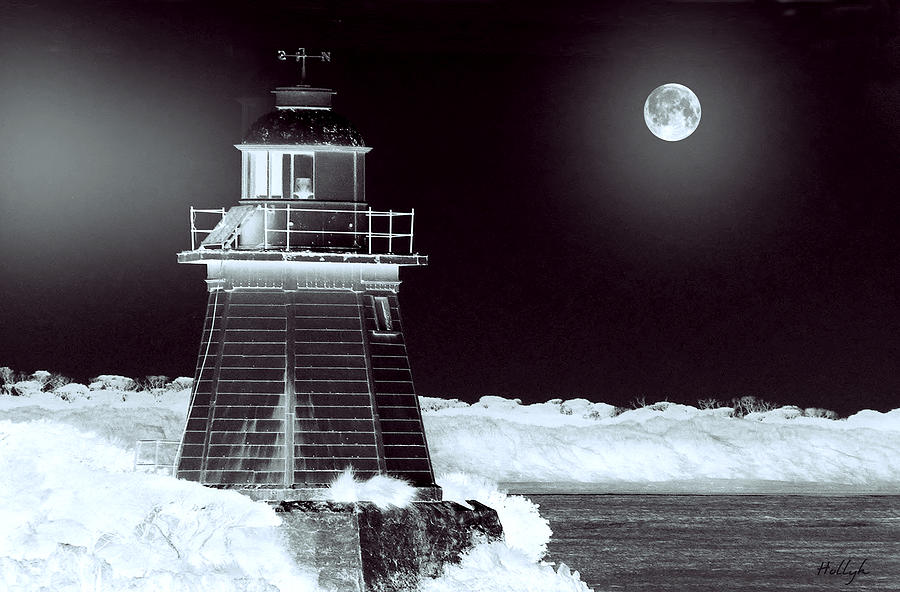This black and white image captures a tranquil winter night, showcasing a small lighthouse standing resolutely amidst a snowy landscape. Positioned near the left edge of the frame, the lighthouse extends from its broad, sturdy base, possibly made of concrete or rock, up to a weather vane adorning its peak. Just below the weather vane, there's an enclosed section with illuminated windows and a surrounding balcony. The structure tapers slightly as it rises, directing viewers' attention toward its functional light.

The right half of the image is dominated by a stark black sky, punctuated by a full moon in the upper right corner. The moon's bright surface, with visible dark areas, casts a grayish halo, creating a striking contrast against the surrounding darkness. Below the moon, a dark, seemingly moving waterway stretches towards the lighthouse, while the snow-covered ground adds a layer of serene stillness to the scene. Despite the absence of houses or other structures, the photograph evokes a sense of quiet isolation, enhanced by the subtle details and atmospheric lighting that suggest it could be a touched-up photograph or an artful combination of a photograph and painting.

Overall, the image presents a rich tapestry of visual contrasts and textures: the cold, still snow, the dark, moving water, the stark, black sky, and the luminous, almost ethereal presence of the moon, all anchored by the steadfast, light-bearing lighthouse.